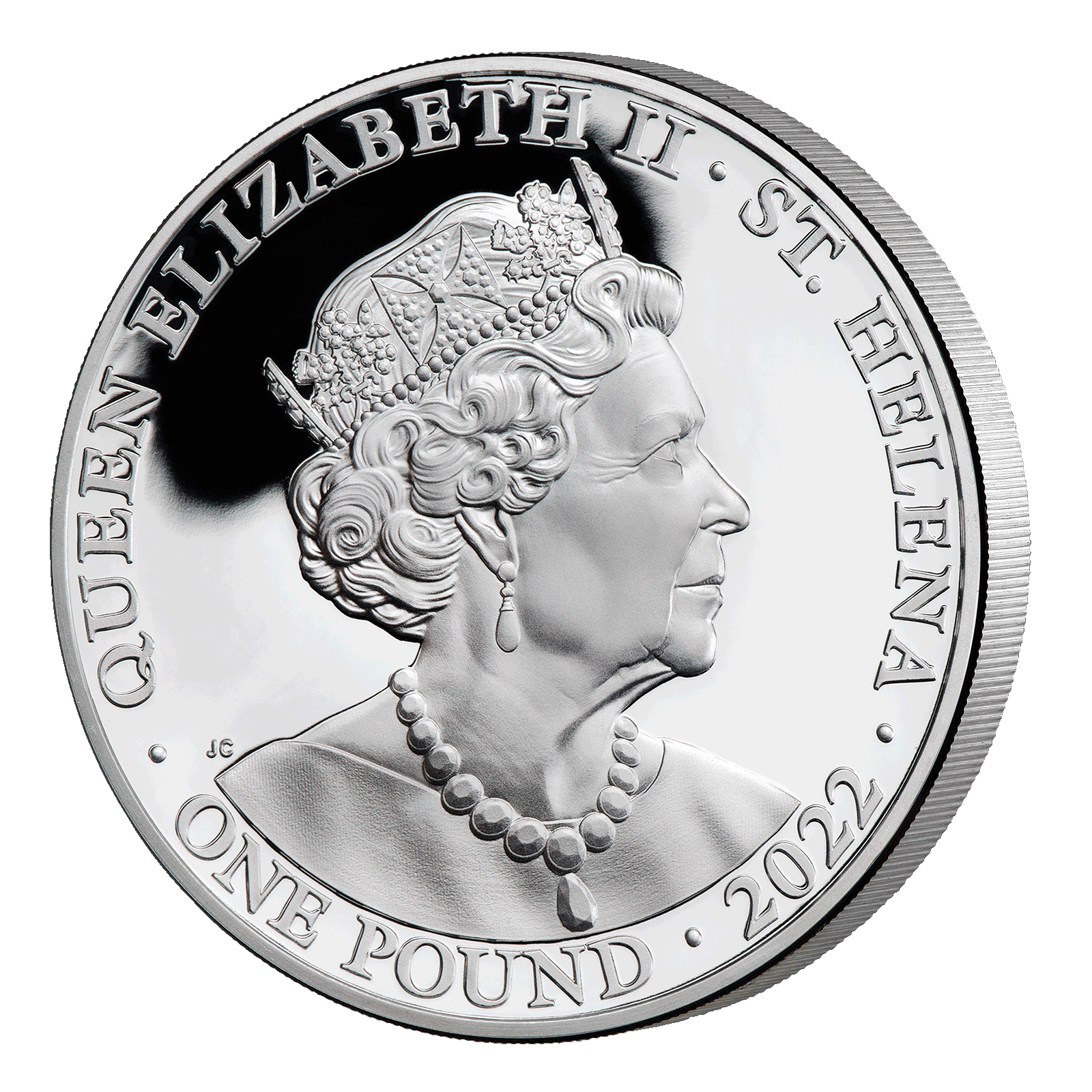The image displays a detailed close-up of a silver British one-pound coin, dating to 2022, from Saint Helena. The coin features an intricately engraved profile of Queen Elizabeth II facing to the right. Her tightly curled hair, adorned with a crown, is captured in remarkable detail, with a string of pearls around her neck and elegant pendant earrings. The text around the edge of the coin reads "Queen Elizabeth II, Saint Helena, 2022, One Pound," arranged in a bas-relief format. The coin is shown at a slight angle, allowing a view of its raised, ridged edge, and the letters "JC" are inscribed to the left of the Queen's portrait, adding to the authenticity of the mint. The image, which appears to be a photographic representation, captures the coin's bright, shiny surface, with subtle shadowing adding depth, particularly behind the crown. Overall, it portrays a beautifully crafted piece that reflects the regal elegance of Queen Elizabeth II.